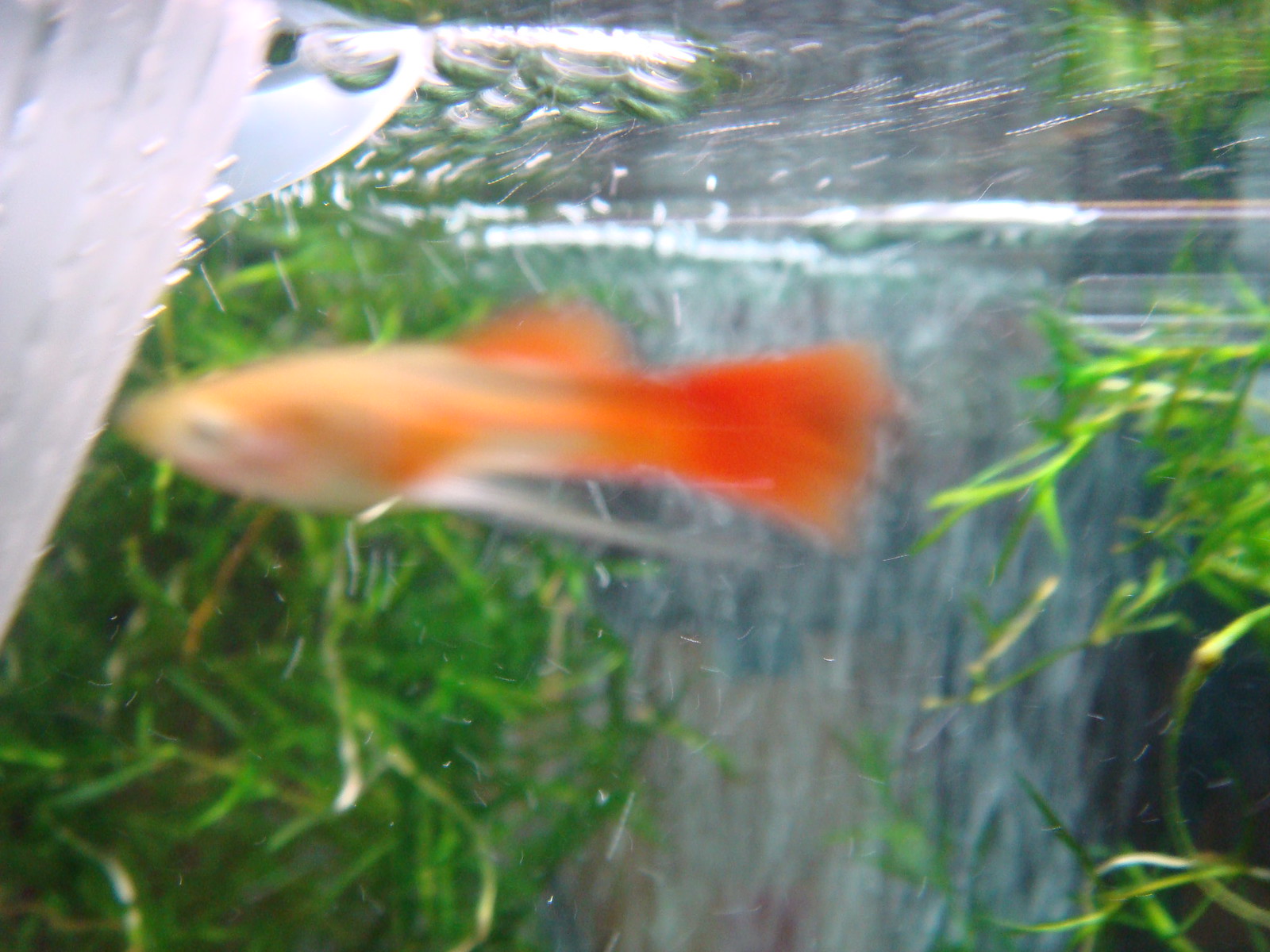The image depicts a blurry, close-up scene of a fish, likely a goldfish, swimming in an aquarium or body of water. The fish's body features a mix of light orange, gold, and silver hues, with a vivid orange tail and fin. The fish appears to be moving towards the left side of the image. Surrounding the fish, the background contains dense greenery on the left, becoming sparser towards the right, where there's a noticeable dark area in the lower right-hand corner. The water seems to create a foggy effect, contributing to the overall lack of sharpness in the image. Additionally, there are indications of a white, mysterious object at the top left edge and possibly a waterfall or wall behind the fish, blending gray and green tones. This composition, combined with the perspective, suggests that the photo was taken either through the glass of an aquarium or while underwater.